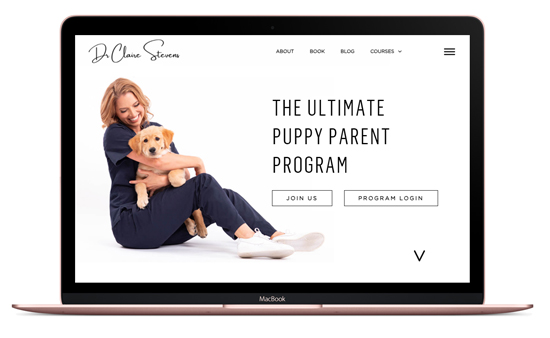In the image, there is a pink MacBook laptop open on a surface. The screen displays a webpage featuring Dr. Claire Stevens, with options for "About," "Book," "Blog," "Courses," and a hamburger menu in the top navigation bar. To the right side of the screen, a person presents the "Ultimate Puppy Pairing Program." Below this presentation, a rectangle button urges viewers to "Join Us." Another rectangular button labeled "Program Login" is accompanied by a down arrow.

On the left side of the image, a person with short hair, dressed in scrubs, holds a small puppy while smiling and looking down at it. The individual is wearing white sneakers. The text on the laptop, displayed in white, highlights various elements, such as Dr. Claire Stevens' featured sections and the Ultimate Puppy Pairing Program. The overall scene captures a warm, professional environment focused on the delightful introduction of a puppy program.